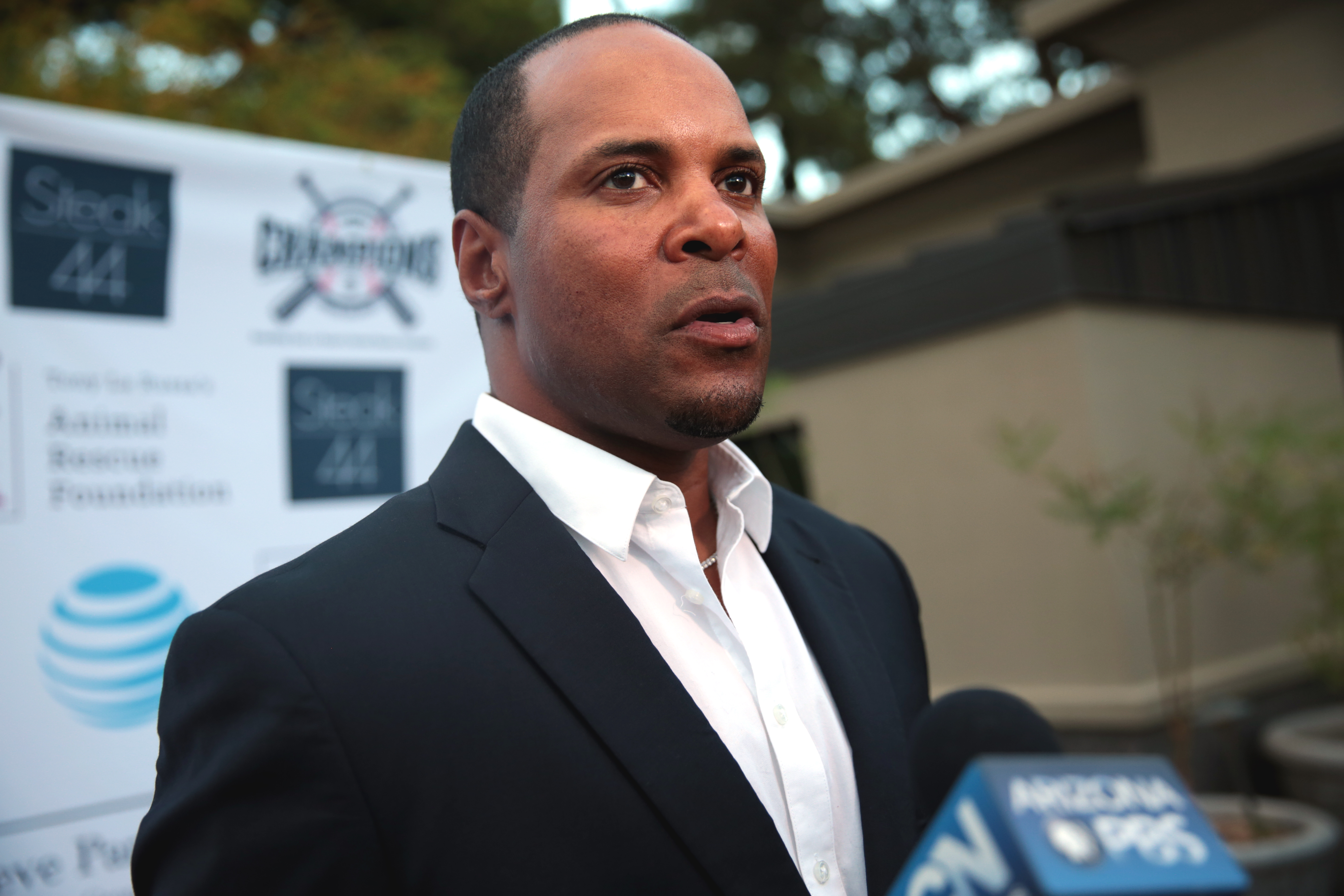In this image, we see a man with very short hair and brown skin, dressed in a black dress suit with a slightly unbuttoned white undershirt. He stands in front of a microphone labeled "Arizona PBS," positioned at the bottom right of the picture. The man appears somewhat puzzled and is looking off to the side, his mouth slightly open and his eyes averted. Behind him, a tan building with brown trim is visible alongside a white backdrop on the left, which displays logos including a blue and white striped circle and solid-colored squares with white text that reads "Stake 44." Additionally, there are some tree tops visible over a wall in the background. The man seems to be giving an interview or answering questions, though he doesn't appear particularly enthusiastic about it.